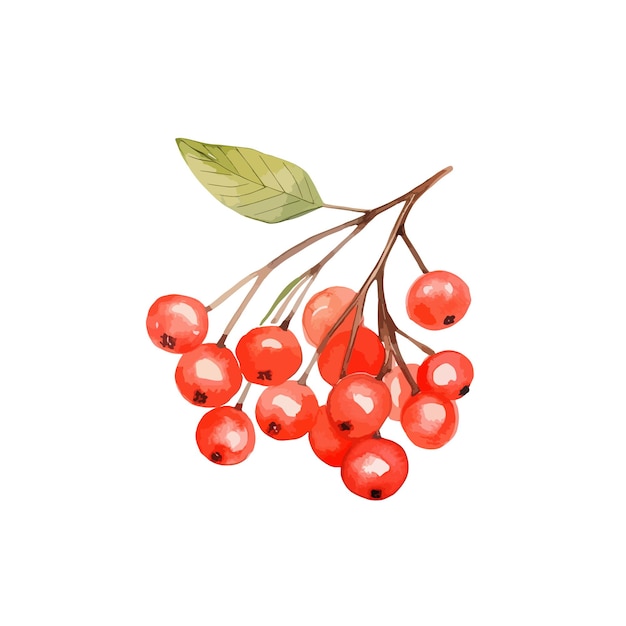The image is a detailed watercolor painting set against a pure white background, depicting a botanical subject with a delicate touch. A thin brown branch enters from the top right, extending diagonally toward the bottom left. As it progresses, the branch lightens to a beige hue and splits off into several finer stems. At the top of the branch, there is a single, nuanced green leaf that exhibits various shades of green—ranging from a grayish lime to light and forest greens. Below the leaf, clustered around the ends of the stems, are around 15 small, glossy red berries. These berries display a range of red hues, including a light salmon color, and feature tiny black spots at their bottom centers, adding a touch of realism and suggesting a reflective, almost glistening quality.